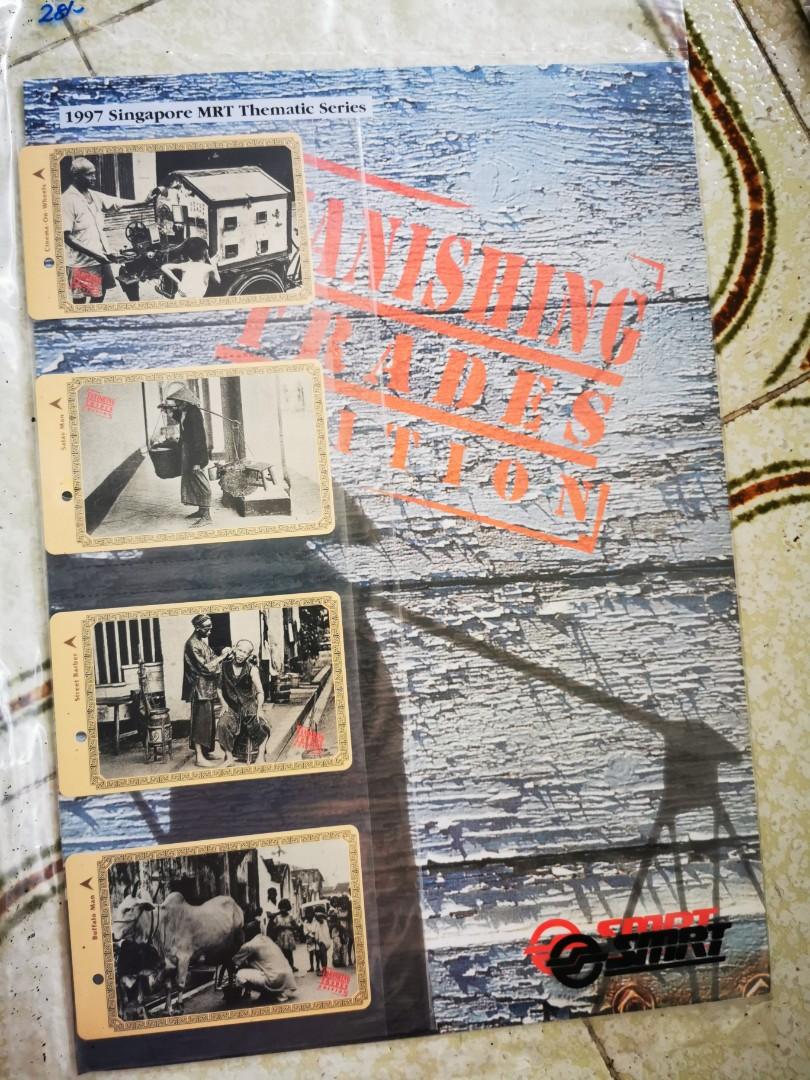This image features a photograph of an old poster set against a weathered, wooden background where the light blue paint is peeling significantly. The poster is titled "1997 Singapore MRT Thematic Series" in a thin banner at the top. Beneath this title, there are four black and white photographs arranged vertically down the left side of the poster, capturing scenes of traditional manual labor in Asia. 

The photographs include: 
1. A man standing next to a small trailer with what looks like a miniature house on top, potentially used for selling goods, with a child nearby.
2. An individual wearing traditional Asian attire, including a straw cone hat, carrying baskets on a pole across their shoulders.
3. A person seated on a stool receiving some kind of service, possibly having their hair cut or ears cleaned, from another person standing beside them.
4. Someone crouching beside a thin, emaciated cow, possibly milking it.

In the lower right corner of the poster, partially obstructed by the photographs, there is text that appears to read "Vanishing Trades", hinting at the poster's theme. Additional unreadable text in a reddish font is also present. The overall scene evokes a nostalgic look at disappearing traditional trades and occupations in Singapore, depicted through a series of evocative photographs and rustic background imagery.